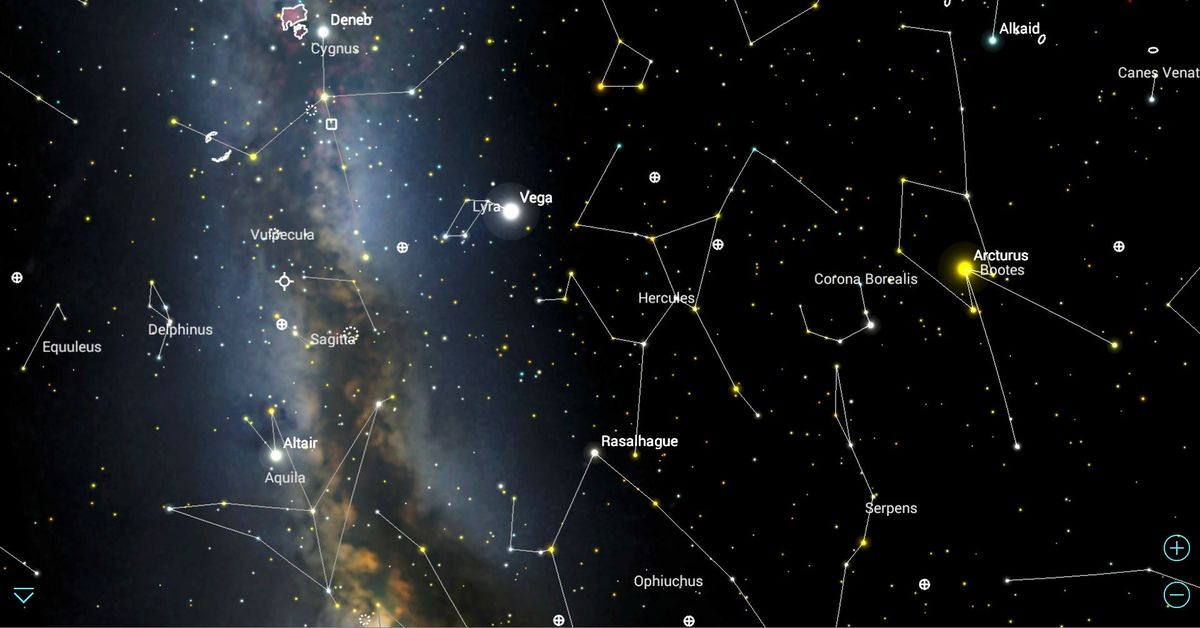This detailed constellation map, viewed through a space telescope, showcases a richly star-studded section of the Milky Way on a dark background. To the left of the image, a galaxy and a nebulous cloud, brighter and illuminated from behind, add depth and intrigue. The celestial display, intricately connected with white lines, features several prominent constellations labeled for easy identification. Starting from the left, notable constellations include Achilles, Delphinus, Deneb, Cygnus, Vulpecula, Sagan, Altair, and Aquila. Towards the right, the map highlights Lyra, Vega, Hercules, Rasselhage, Ophiuchus, Corona Borealis, Serpens, Alkaid, Arcturus, Bootes, and Canes Venatici. The far-right side of the image is characterized by a darker, denser scattering of tiny stars, contrasting with the luminous center-left region.